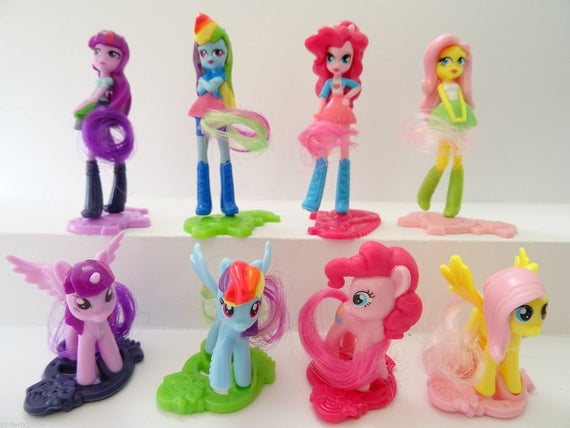The image showcases a bright and clear close-up of a toy collection displayed on two rows against a white background. The bottom row features four My Little Pony characters, each with combable fake hair on their manes and tails, and wings like a unicorn. The ponies come in distinct colors: a purple pony on a purple base, a light blue one with rainbow-colored hair on a green base, a light pink pony with darker pink hair on a dark pink base, and a yellow pony with pink hair on a matching pink base. Above each pony is a corresponding human-like figurine, mirroring the colors and features of the ponies beneath them. These figurines, resembling Bratz dolls, are all female with colored hair and dresses, complete with tall boots. The purple, light blue, pink, and yellow human figures perfectly match their respective My Little Pony characters below, creating a cohesive and visually appealing display.